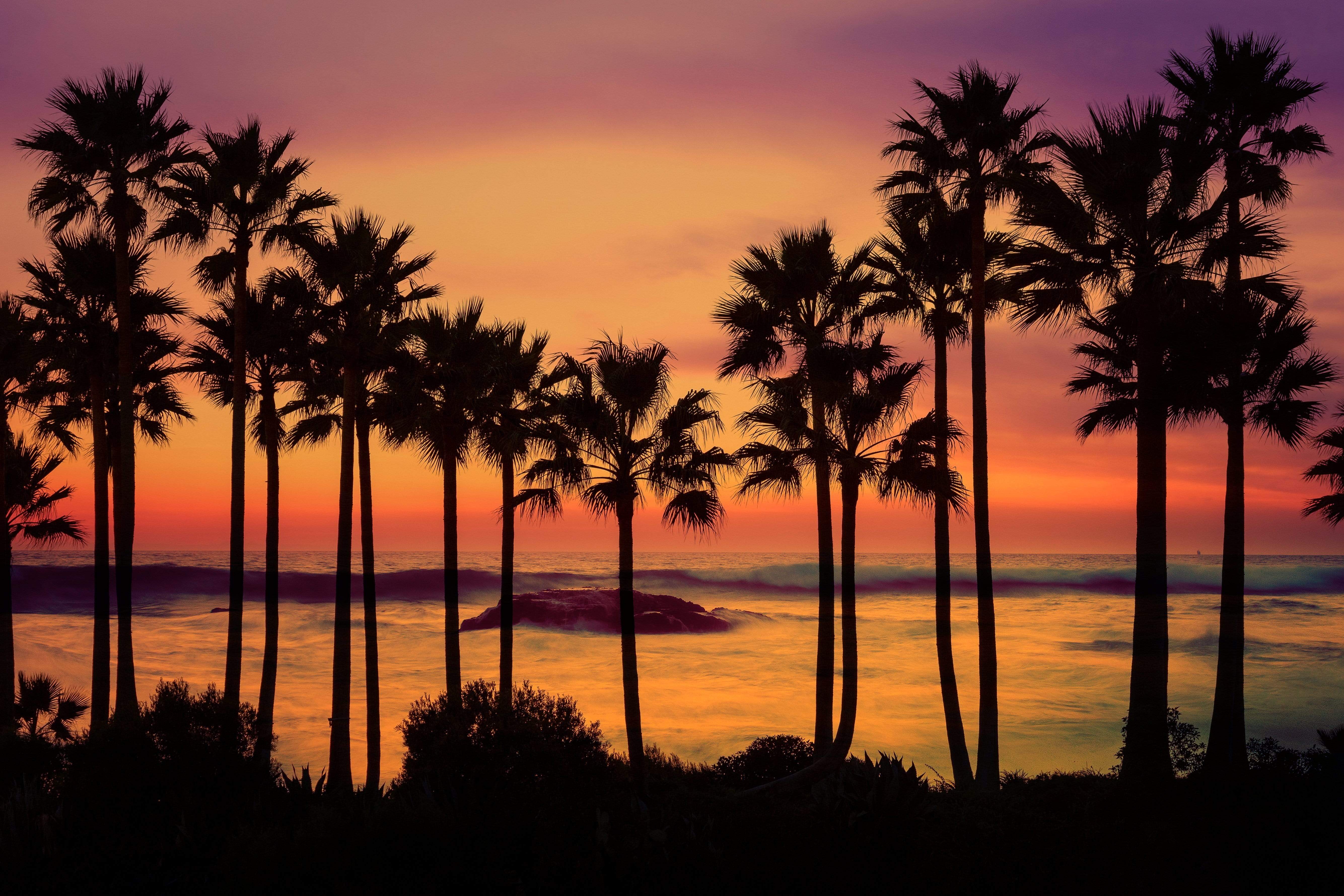This stunning tropical sunset scene features a vibrant sky painted with deep oranges, purples, and yellows. The sun has already dipped below the horizon, casting the entire landscape into beautiful silhouette. Waves gently roll towards the shore, and a small rock protrudes from the otherwise smooth beach surface. Framing the scene is a dense row of palm trees, stretching from the left to the right, their silhouettes stark against the colorful backdrop. Beneath the palms, shadowed vegetation adds texture to the foreground, leading the eye towards the dark, serene expanse of water. This is the kind of photo that would grace a Hawaii hotel brochure, inviting travelers to experience paradise.